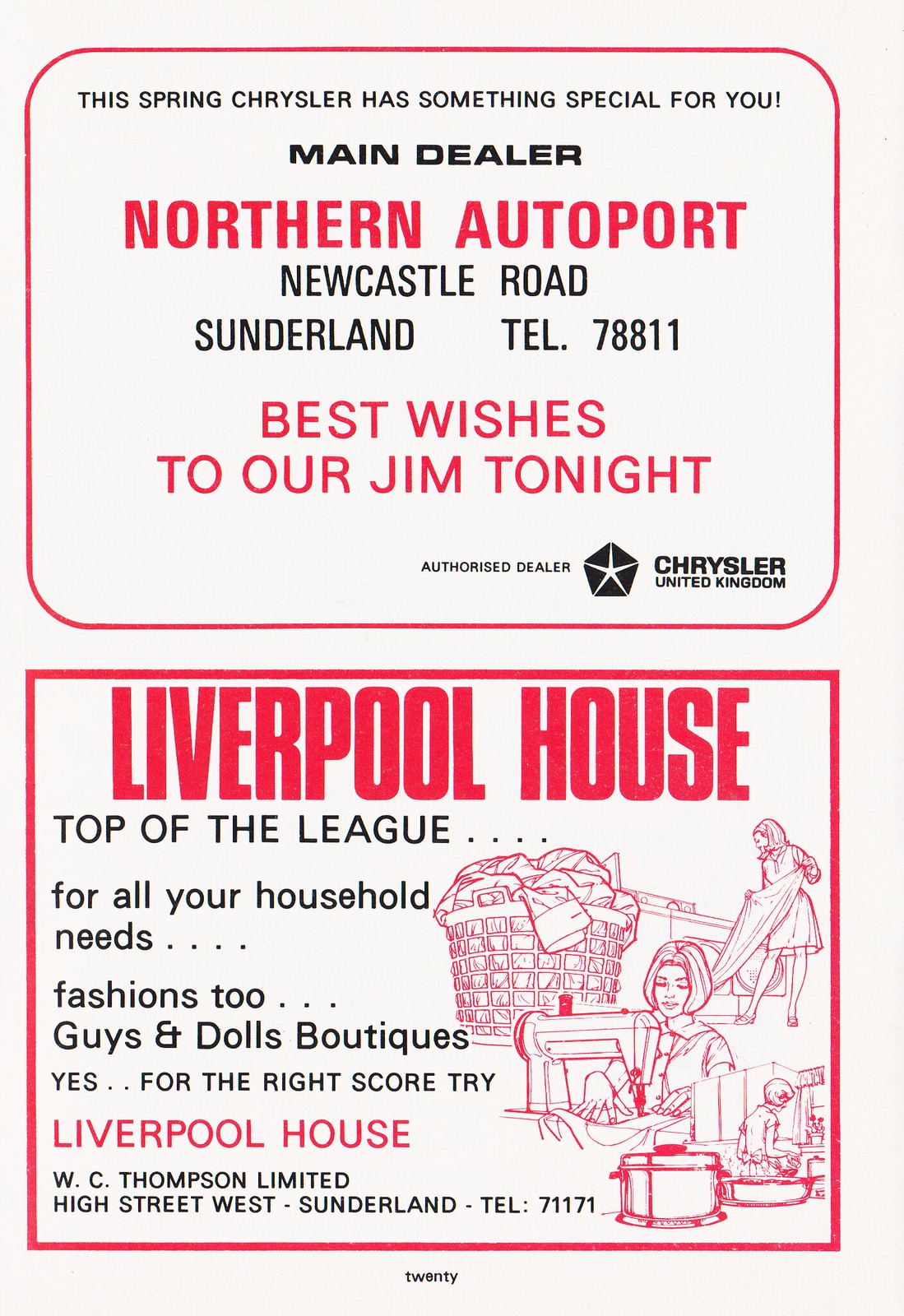The image appears to be a page from an old magazine, specifically page 20. It features two advertisements, stacked one above the other. The top advertisement promotes Chrysler, featuring the text "This Spring Chrysler has something special for you" in black ink. Below this, the ad highlights "Main Dealer Northern Auto Port, Newcastle Road, Sunderland" with the telephone number "78811" in black ink as well. The phrase "Best wishes to our gym tonight" is displayed prominently in bold red letters inside a red-bordered box. The phrase "Chrysler United Kingdom" with a small logo appears on the right-hand side.

The second advertisement, separated by a red outline, is for Liverpool House. The heading "Liverpool House" is in bright bold red letters followed by "Top of the league for all your household needs, fashions to guys and dolls boutiques" in black ink. On the right-hand side of this ad, there are illustrations of women engaged in household activities such as doing laundry, using a sewing machine, and cooking with pots on a stove. A large laundry basket filled with clothes is also depicted. The slogan "Yes for the right score, try Liverpool House" is written in red ink. The name "WC Thompson Limited, High Street West, Sunderland" and the telephone number "71171" appear at the bottom. Both ads primarily use red and black ink.